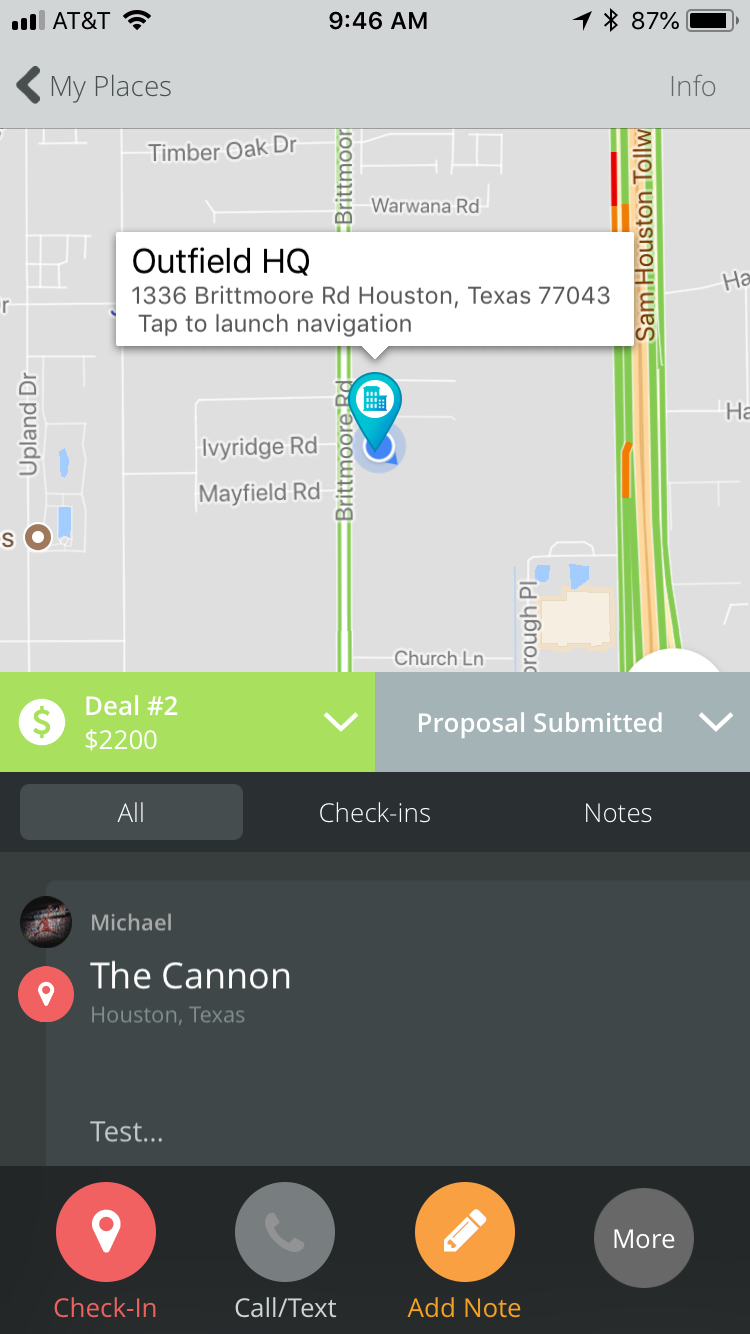The image displays a navigation interface from a GPS-based app. The map prominently highlights "Outfield Headquarters," located at 1336 Britmore Road, Houston, Texas, 77043. Below the map section, there is a prompt that reads "Tap to launch navigation."

Beneath this prompt is a panel divided into two sections. The left side of the panel shows "Deal Number 2, 2200" within a green rectangle. To the right, "Proposal Submitted" is displayed inside a grey rectangle, though its exact context—whether an advertisement or a sales-related instruction—is unclear.

Further down the screen, several options are available, including "All Check-ins" and "Notes." An icon displays a user referred to as "Michael," with the location marked as "The Cannon, Houston, Texas." It appears that Michael is in the process of typing "test..." in a window.

At the bottom of the screen, there are multiple action buttons: a red "Check-in" button, a grey "Call/Text" button, an orange "Add Note" button, and another grey circular button labeled "More."